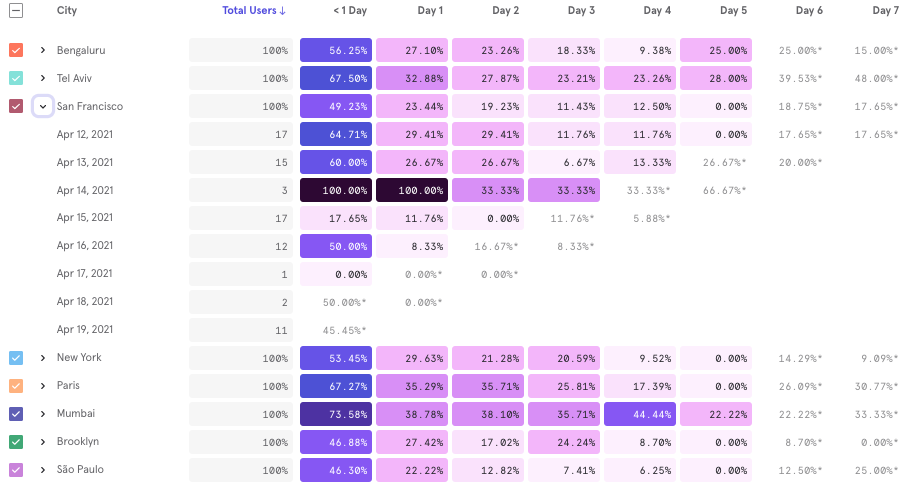This web page displays a comprehensive, color-coded dataset. Each individual box contains specific data, predominantly percentages, and is uniquely color-coded: bright blue, purple, light purplish pink, black, and gray. Along the left margin, the header "City" appears in gray text, with a list of cities below it, including Bengaluru, Tel Aviv, San Francisco, New York, Paris, Mumbai, Brooklyn, and Sao Paulo. Across the top, a bright blue header labeled "Total Users" is prominently displayed, followed by a vertical column of data categories such as "One Day," "Less Than One Day," "Day 1," "Day 2," "Day 3," "Day 4," "Day 5," "Day 6," and "Day 7." Each city's corresponding data for these days is shown in the color-coded boxes. Notably, San Francisco has additional entries for dates in April 2021, suggesting that a drop-down menu has been clicked to reveal this extra information.